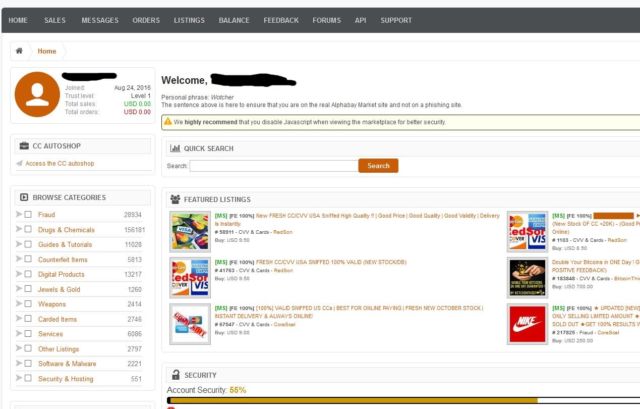The screenshot depicts the homepage of a suspected dark web marketplace named "Alpha Bay Market." The upper section of the page features a black navigation bar with various tabs including Home, Sales, Messages, Orders, Listings, Balance, Feedback, Forums, API, and Support. To the left, a sidebar lists categories such as Browse Categories, Fraud, Drugs and Chemicals, Guides and Tutorials, Counterfeit Items, Digital Products, Tools, and Goals.

A welcome message, partially obscured for privacy by the term "watcher," is displayed. In very small text, the website reassures users that they are on the legitimate Alpha Bay Market and not a phishing site. It also advises viewers to disable JavaScript for enhanced security. This confirms the site is part of the dark web, engaging in illegal or dubious activities.